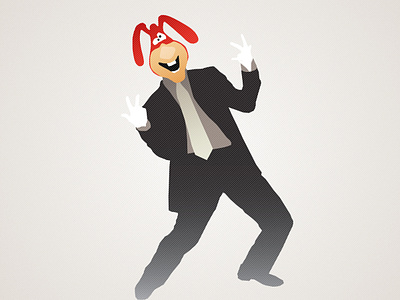The image depicts a cartoonish character set against a gradient background, transitioning from gray to white. The character is dressed in a formal black suit with a gray shirt, a white tie, and black shoes. They are wearing white gloves and are captured in a dynamic pose, leaning back with their knees bent and holding up three fingers on each hand.

The character’s head is distinctive and blends elements of both a donkey and a mask-like appearance. The face is predominantly brown and orange, with an exaggerated smile revealing large front teeth and smaller lower teeth. The eyes are white and googly, protruding through a red top portion of the character’s head, which features long, floppy ears hanging down. The nose is large and prominent. The entire scene is playful and whimsical, evoking a sense of familiarity yet is difficult to identify specifically with any known character or franchise. No text accompanies the image.